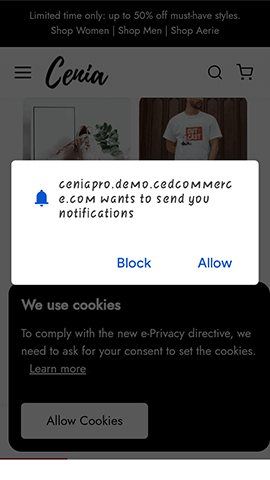The image showcases the homepage of a website named CENIA, stylized as "CENA." The top section features a promotional banner on a black background with bold white text announcing a "Limited Time Only: Up to 50% Off on Must-Have Styles." Below the banner, there are options to "Shop Women's Line," "Shop Men's Line," and "Shop AERIE." 

The website's header includes the name "CENIA" along with icons for a shopping cart, a magnifying glass for search, and a pull-out menu represented by three horizontal lines. The main page is partially visible, showing two photos of featured items.

A semi-transparent gray overlay covers the entire background, indicating an active modal. At the center of the screen, a white pop-up window reads, "CENApro.demo.C-E .com wants to send you notifications." The options "Block" and "Allow" are prominently displayed inside blue buttons. Next to this message, there's a blue bell icon.

Below the notification request, the pop-up further informs users about cookie usage in compliance with a new e-privacy directive. The text reads, "We use cookies to comply with a new e-privacy directive, we need to ask for your consent to set the cookies." The phrase "Learn More" is underlined, indicating a link, and there is a white button with black text that says "Allow Cookies."

The detailed information and interactive elements make it clear that this website is providing a secure and user-friendly shopping experience while adhering to privacy regulations.